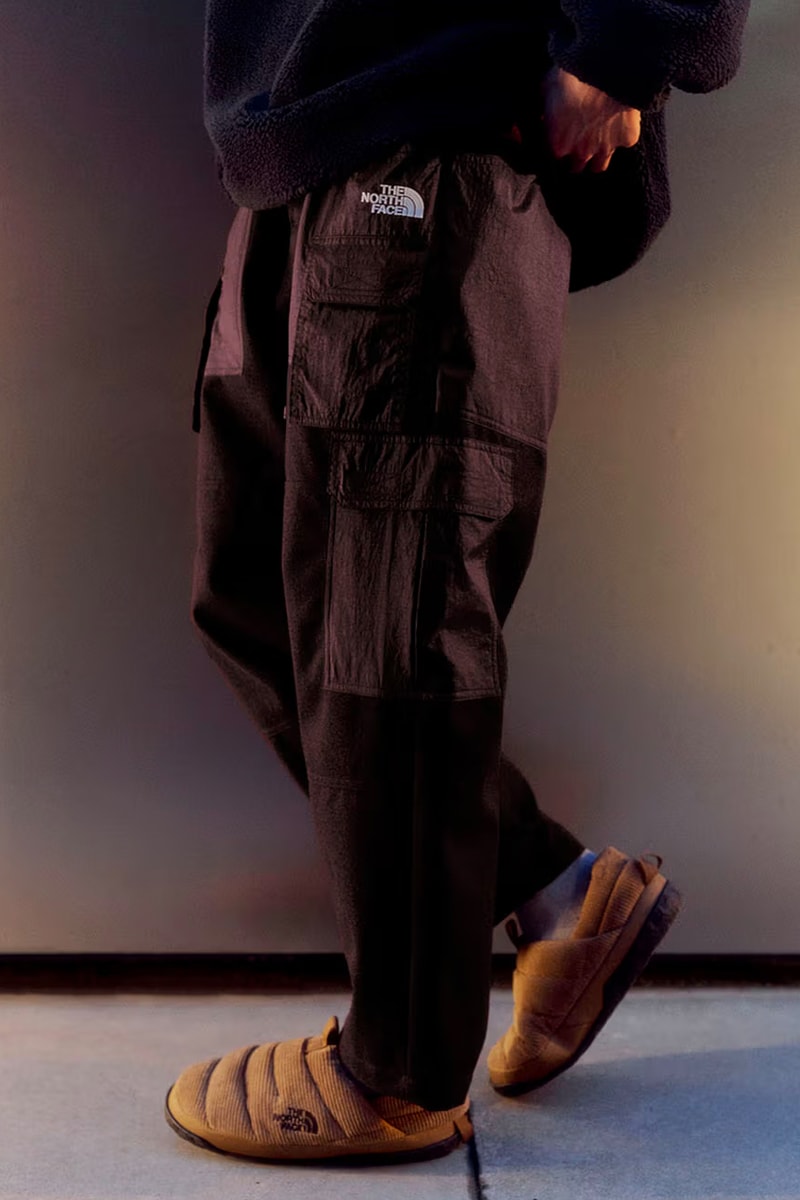In this advertisement-themed photograph, a model is captured from the waist down, emphasizing the stylish black North Face cargo pants designed for outdoor use. He's casually poised against a plain, grayish, or beige background with a semi-white or ceramic-tile floor beneath him. The model, mid-walk and mid-stride, adds a dynamic element to the image. His attire includes cushy North Face slippers, tan in color, paired with white socks. He leans on his left foot while his right foot is tipped, contributing to a relaxed, effortless vibe. The image is sterile and minimalistic, drawing attention to the functional yet fashionable cargo pants adorned with a white logo on the upper pocket.